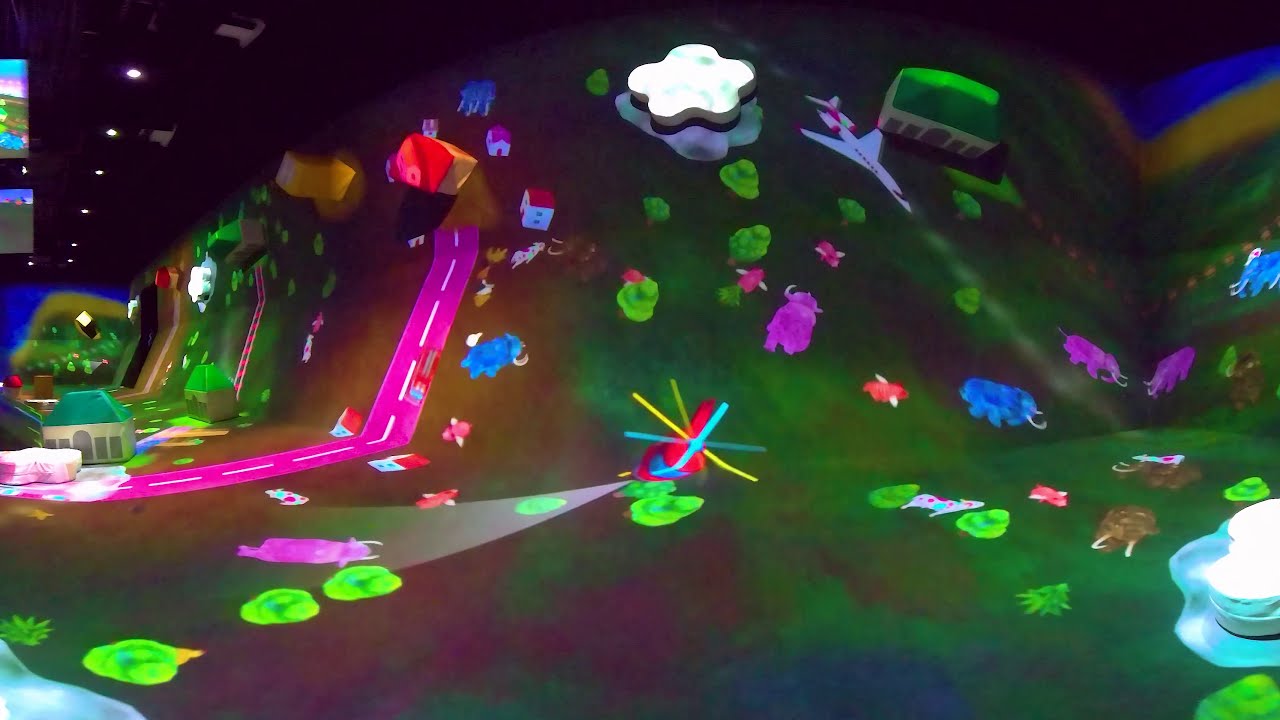The photograph captures what appears to be an animated scene set within a room, suggesting a possible projection or digitally created display. The focal point is a vibrant landscape featuring a green ground that slopes up into a mountainous terrain. On the left side, a prominent pink road with white lane stripes cuts through the scene, meandering towards the center and ascending into the mountain. Scattered throughout the landscape are various objects including blue elephants, green flowers, bushes, and trees, adding a whimsical nature to the setting.

Positioned above, a red cartoon helicopter with blue and yellow propellers hovers in the air, alongside a cloud and a white airplane located in the top right corner. The colors in this image are vivid and diverse, with hues of black, white, yellow, light blue, pink, purple, tan, and various shades of green and blue peppering the scene. The arrangement of elements appears random, with no particular focus, lending a chaotic yet charming feel to the image. The environment includes smaller structures such as homes and a building, enhancing the realistic yet fantastical element of the scene.

Ambient light from the real room can be seen in the upper left corner of the image, indicating that the animated scene is being viewed within a physical space. The overall image, though slightly distorted, is rich in detail and color, creating an engaging and imaginative visual experience.